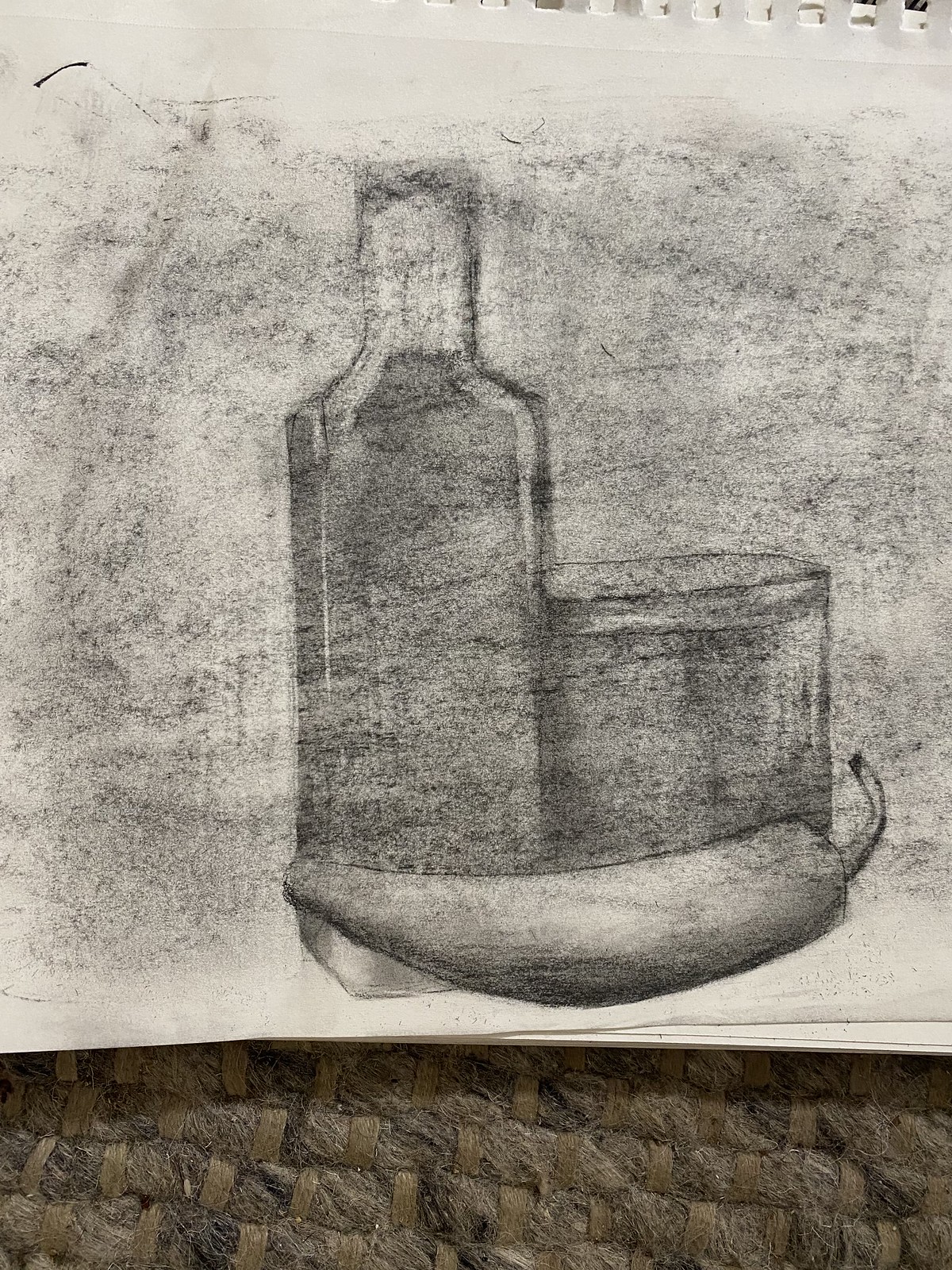This image is a detailed photograph of a charcoal sketch on white notebook paper that has been torn from a spiral-bound notebook, evidenced by the jagged, torn edges at the top. The sketch itself is an expressive still life, entirely rendered in shades of gray and soft, hazy charcoal. The subject of the drawing includes a tall, square-shaped glass bottle—possibly resembling a gin bottle—and a low, round glass container to its right, which might be filled with liquid. In the foreground, a pepper—appearing to be a jalapeno—is positioned horizontally, with its pointed tip facing left and its stem pointing right. The background of the sketch features rough charcoal shading, enhancing the contrast and providing depth to the still life arrangement.

This paper with the sketch appears to be placed atop additional pages or possibly the notebook itself, which are slightly visible along the lower edge. Beneath the paper, there's a woven natural material that resembles a lightly-colored jute rug or quilt, visible through its tan, brownish stitching. The background material and the rough charcoal shading lend a textured and somewhat rustic feel to the entire setup.